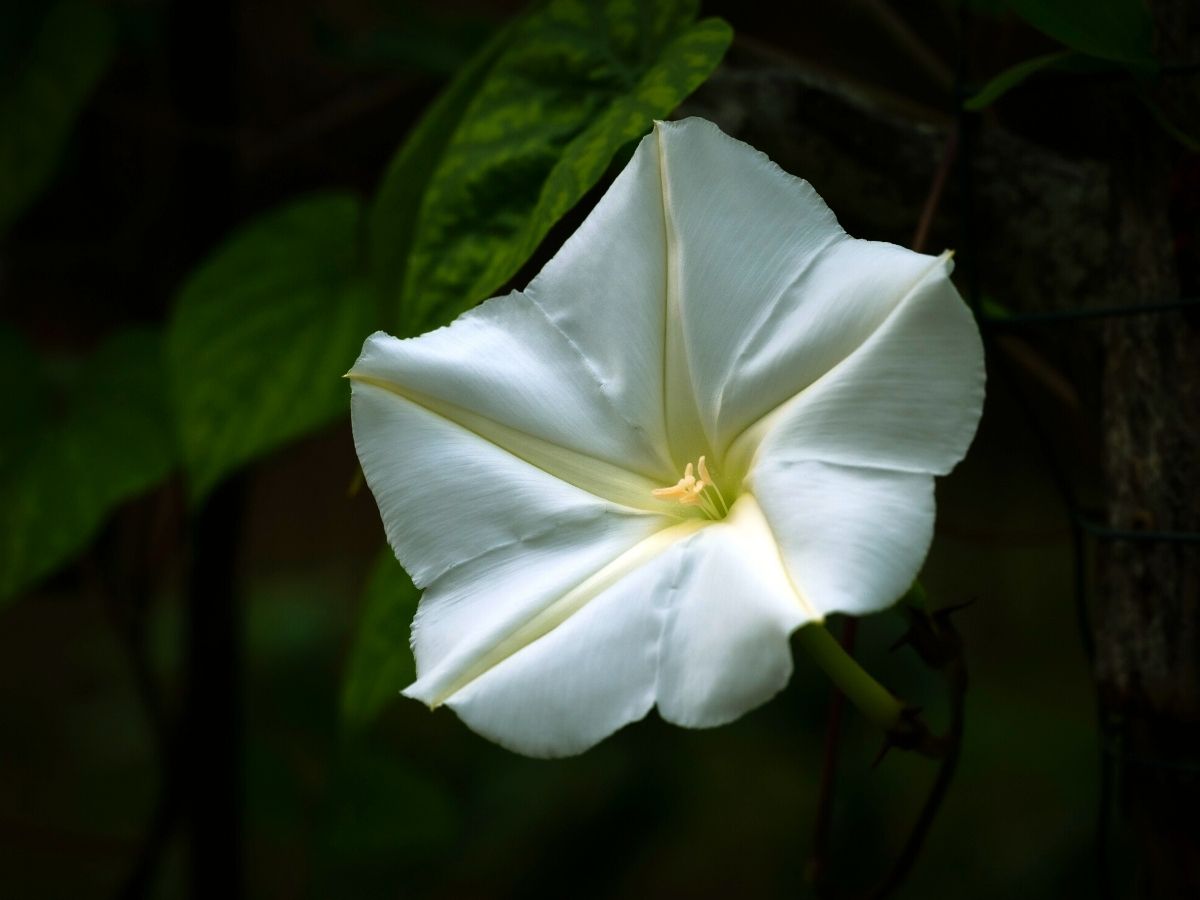This is a macro, close-up, high-resolution photograph of a striking white morning glory flower, showcased in intricate detail. The flower, prominently positioned at the center of the image, has a star-shaped form with five white petals that subtly merge, each displaying a delicate, pinstripe texture. Each petal is marked with a faint yellow line running from the tapered edges toward the flower’s pale yellow center. In the middle, a cluster of yellow stamens stands out vividly. The flower's green stem extends into a vine, partially visible amidst the dark, out-of-focus background which adds depth and contrast to the image. Several green leaves, primarily located in the upper left-hand corner, offer added texture and visual interest, their veins discernable despite the dim lighting conditions that suggest the photo might have been taken at night.